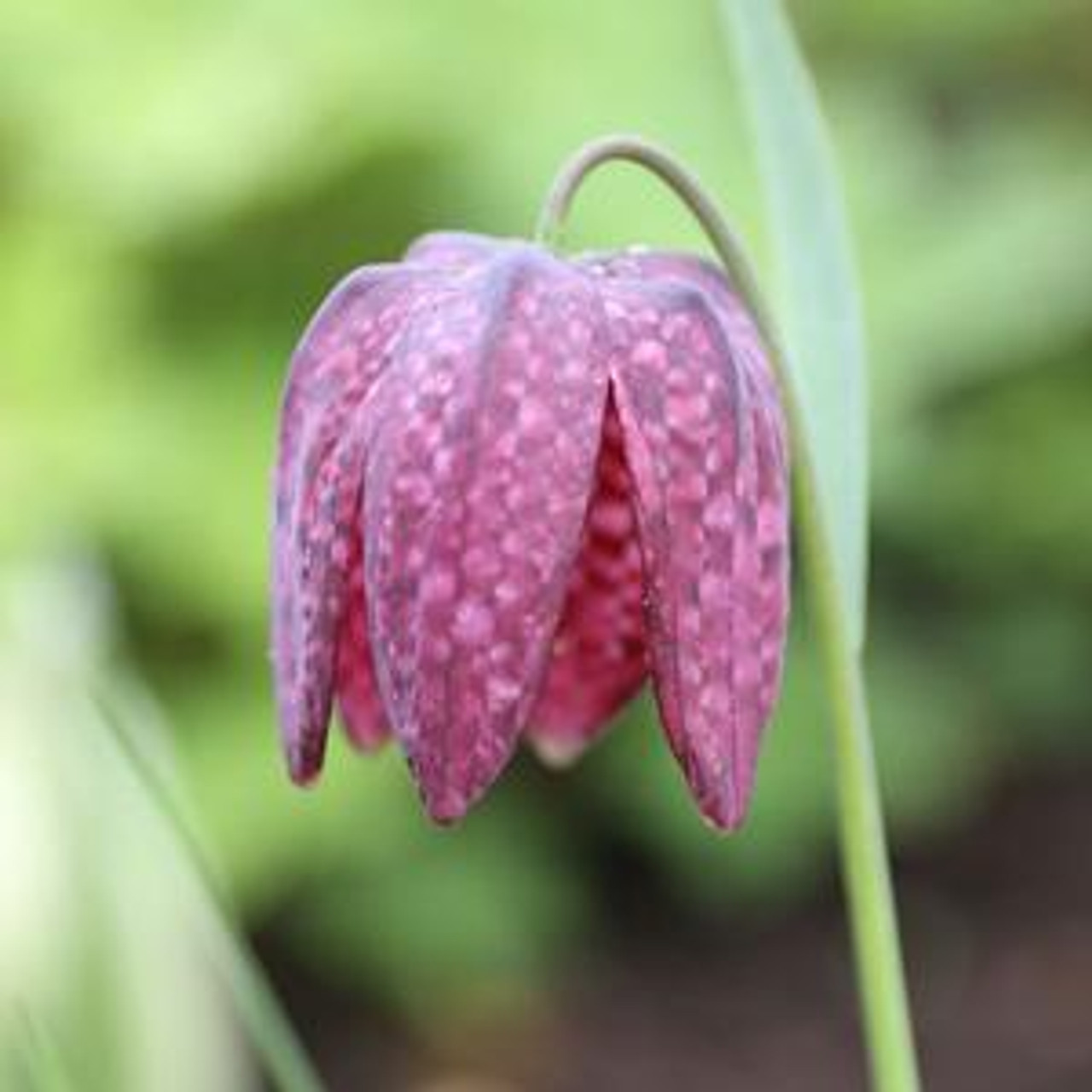The image showcases a high-definition close-up of a vibrant pink Meleagris flower, captured by a nature photographer in bright, daylight conditions. The flower, adorned with distinct dotted patterns on its petals, bends gracefully downward. Its lush green stem, along with a single leaf, adds contrast and depth to the composition. The background, though blurred to draw attention to the flower, reveals a hint of greenery and possibly brown soil, suggesting an outdoor setting abundant with plants or grass. The overall clarity of the image is exceptionally bright and sharp, emphasizing the intricate details of the Meleagris while providing a serene, natural backdrop.